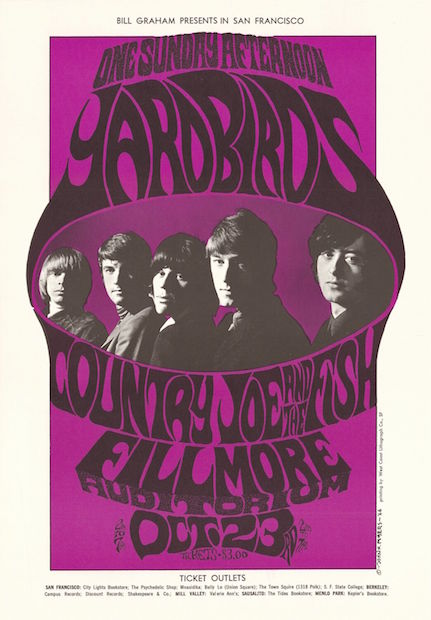This is a detailed, psychedelic concert poster advertising a performance at the Fillmore Auditorium in San Francisco. Framed against a white background, a large purple rectangle dominates the poster, inside which it says "Bill Graham Presents" at the top. Emphasizing a trippy, spaced-out lettering style typical of the era, the date "October 23rd" is noted, indicating a Sunday afternoon event. The headline acts are the Yardbirds and Country Joe and the Fish, with the names appearing in large, squiggly letters. Centrally featured within an oval, there's a black-and-white photograph of the Yardbirds band members, their hair shaded darker and styled in late 60s and early 70s fashion. Around the edges, the poster lists several ticket outlets.